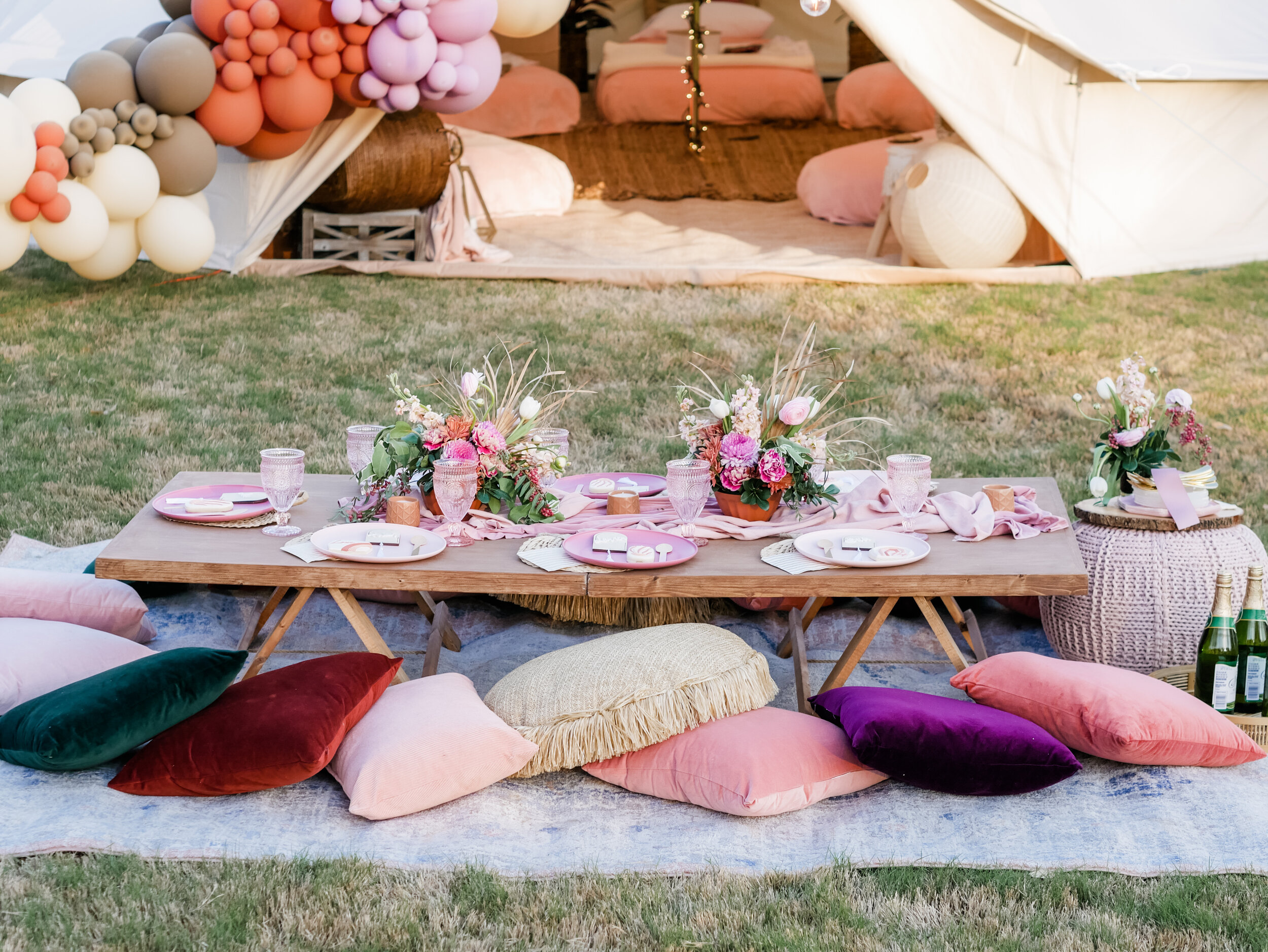In this picturesque outdoor setting, a cozy picnic scene is showcased on a lush green lawn. Centered on a large mat, a small brown picnic table is surrounded by an array of colorful cushions in shades of purple, pink, yellow, and green, inviting guests to sit and relax. The table is meticulously set with plates and cups, some containing delicious pastries and various drinks. Adding a touch of elegance, two flower pots with beautiful bouquets adorn the center of the table, alongside two bottles of wine resting in the lower right corner. A large picnic basket is also present. In the background, a whimsical tent decorated with balloons in hues of purple, green, orange, brown, and white stands tall. Inside the tent, there are comfortable beds, creating a serene and inviting atmosphere perfect for a tranquil gathering.